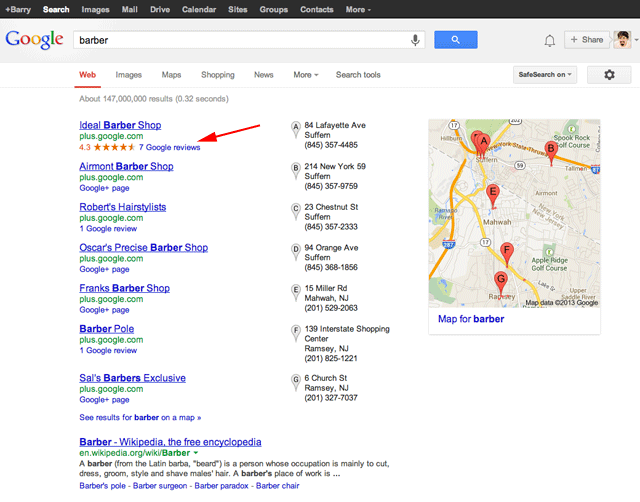This is a detailed screenshot of the Google search page. At the top, a black navigation bar spans across the screen, displaying various Google services including "+Berry," "Search," "Images," "Mail," "Drive," "Calendar," "Sites," "Groups," "Contacts," and "More." Below the black bar, a light gray bar houses the iconic Google logo on the left and a central search bar that contains the term "barber." To the right of the search bar is a blue search button. Adjacent to this button are additional icons: a bell notification icon, a "+Share" button, and a profile picture with a drop-down menu. Following this, another navigation menu displays options like "Web," "Images," "Maps," "Shopping," "News," "More," and "Search tools." In the main body of the page, there are eight search results with blue hyperlinks. To the right, a small map is visible featuring red pins that mark specific locations.